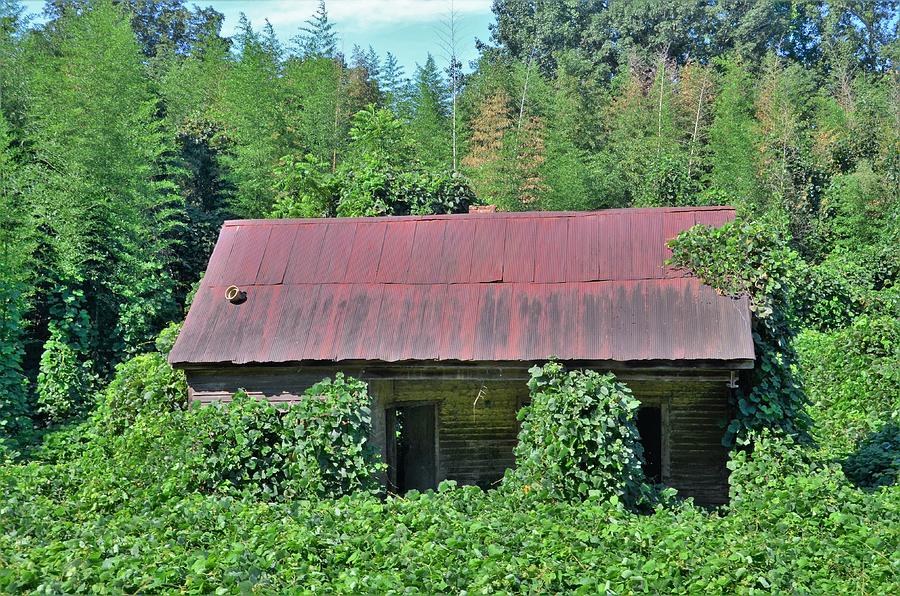This image depicts an abandoned, rustic wooden shack with a rusted tin roof, clearly built before 1900, and possibly located in Georgia, amidst the deep southeastern woods. The structure is being overtaken by lush, wild overgrowth, primarily kudzu, which engulfs the entire front of the shack, heaping over what was once porch posts, the door, and the window. The kudzu even extends to the roof, covering portions of it. The roof itself has large, rectangular rusted tiles and displays black streaks along its bottom half. A little brick chimney can be spotted at the back of the house, and there's an unusual sight of a pot placed on the roof. To the left side of the shack, the vines are predominantly overgrown, casting shadows over the lone partially open door. 

The shack is surrounded by a dense forest patch of tall, likely invasive bamboo, stretching upwards behind the building. Beyond the bamboo, the presence of a natural hardwood forest is evident, creating a backdrop of towering trees, some brownish-yellow in color. While the right side of the image shows more of the oppressive, thick forest growth, the left side opens up to a glimpse of a clear, blue summer sky dotted with clouds. It's a serene yet desolate scene showcasing the relentless reclaiming force of nature over human creation.